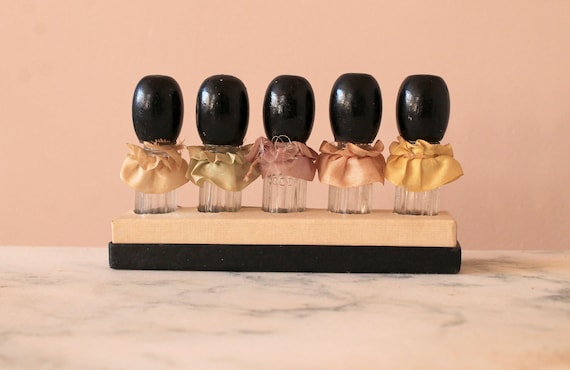This color photograph, likely taken indoors with artificial lighting, features a clear, staged setup with no border. Centered in the image is a homemade craft consisting of a wooden holder with a plastic base. This rectangular holder, wood-colored with a black-painted bottom, rests on a marble-like countertop characterized by black streaks. The background is a pinkish beige wall.

The holder has five round holes, each containing a narrow, cylindrical glass vial. These clear glass vials are adorned with frilled fabric circles near their black-painted, large, oval-shaped lids that resemble shiny, reflective olives. Each vial's frill comes in different colors, including mauve, green, purple, peach, and gold. The purpose of these vials is unclear, though they could possibly be used for storing herbs or perfumes. This meticulously arranged setup features no people, animals, or text, further emphasizing the craft as the focal point.